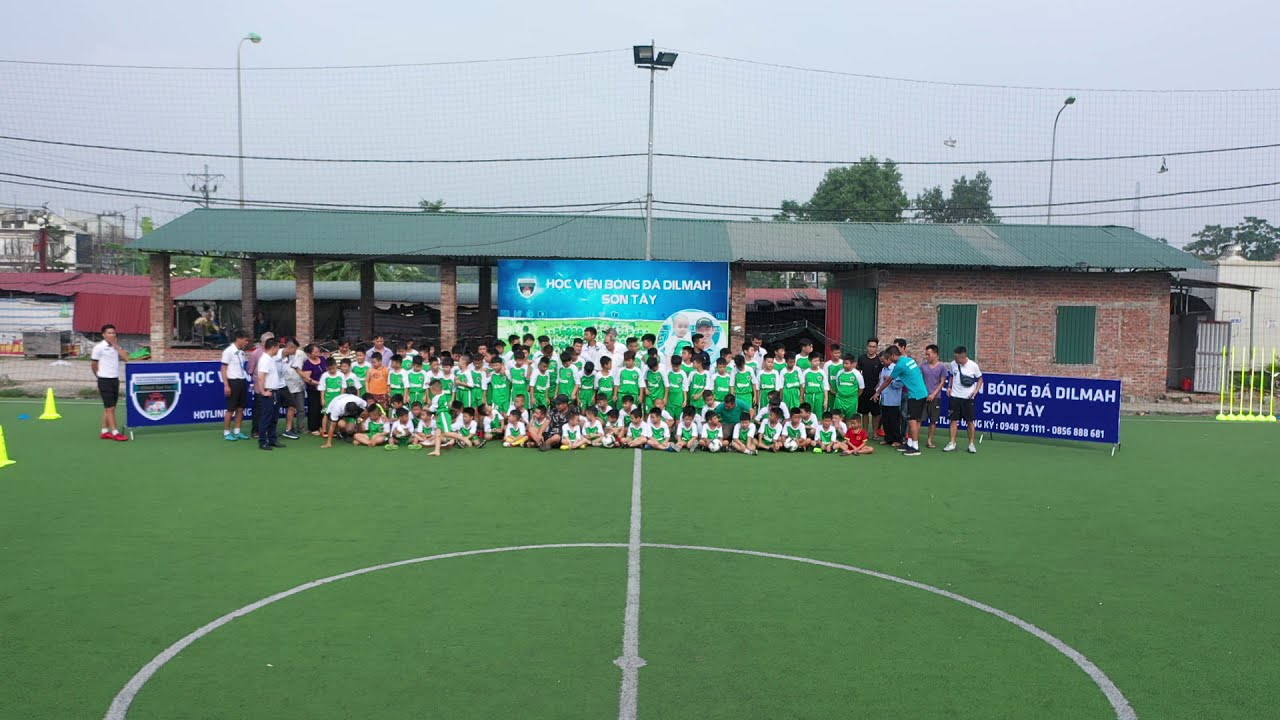In this detailed and vibrant photograph, a group of young children, clad in matching green and white sports jerseys and pants, are arranged meticulously for a team photo in front of a brick outdoor patio with a green metal roof. The children are positioned in two rows: one standing at the back and a smaller group sitting in the front on a field of green turf marked with white lines, resembling a soccer or sports field. Flanking the cluster of children are adults in casual clothing; one on the right, wearing a teal shirt and black shorts, is pointing at something on the ground, while another on the left, dressed in a white shirt, black shorts, and red shoes, stands near two yellow safety cones. Additional adults in various attire, including a white shirt with a black bag, surround the children. Prominent blue signs with stark white lettering in a foreign language stand on both sides of the group and another similar sign hangs on the brick patio's roof behind them. The background reveals two green-shaded windows, brick pillars supporting the patio roof, a net attached to a central light post stretching across the scene, and distant buildings peeking above the roofline against a hazy gray sky.